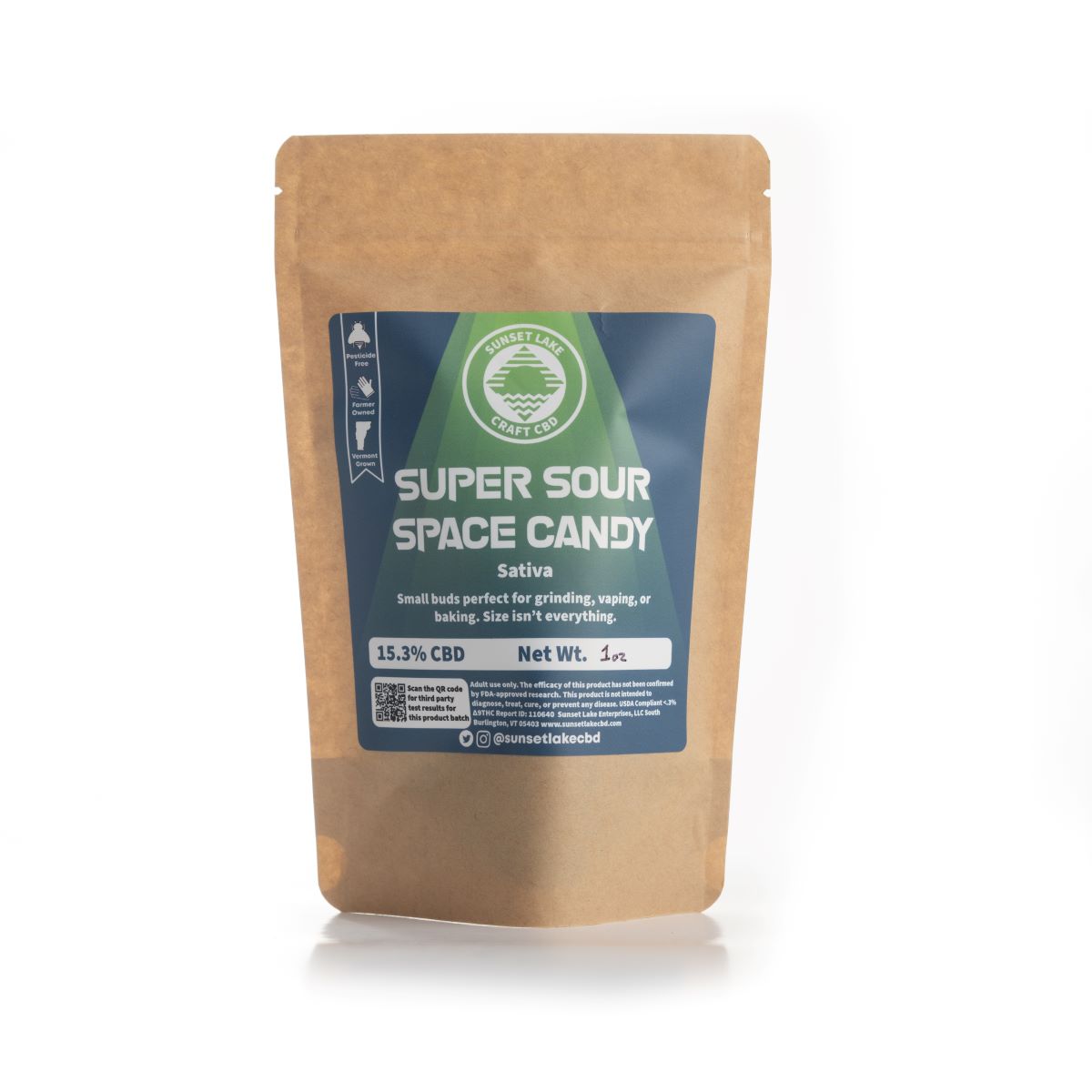The photograph features a resealable brown paper pouch with a tear strip at the top, resembling flexible, multi-layer packaging. A prominent blue label on the front showcases whimsical graphics, including a green beam reminiscent of a flying saucer's tractor beam and white text. The product is "Super Sour Space Candy" by Sunset Lake Craft CBD, described as sativa small buds perfect for grinding, vaping, or baking, with the tagline "Size isn't everything." The label details its 15.3% CBD content and a net weight of 1 ounce. Additionally, it includes a QR code, the Sunset Lake Craft CBD logo—which depicts a sun setting over a lake or ocean— and social media icons for Twitter and Instagram. There is also a disclaimer noting that the product is intended for adult use only and has not been evaluated by the FDA to diagnose, treat, cure, or prevent any disease.